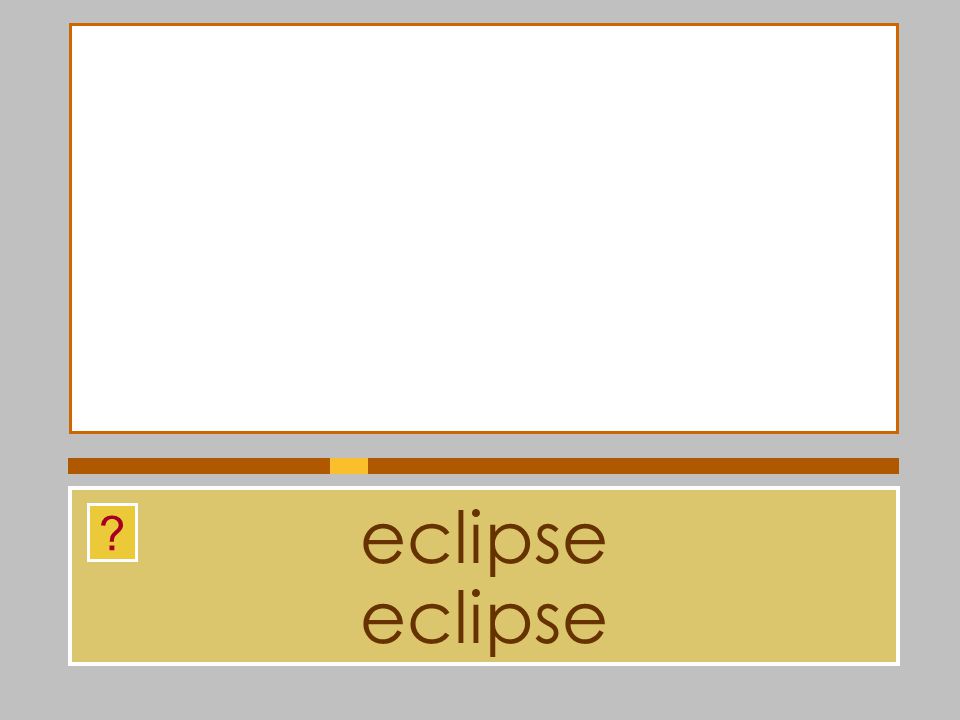The image depicts a simple yet incomplete slide design with a wide vertical rectangle format and a gray background. Centrally positioned within this layout are two prominent horizontal rectangles. The top rectangle is a substantial white box with a thin brown border but no text or imagery inside. Beneath this is a brown horizontal stripe extending across the width of the slide, featuring a small gold rectangle positioned about a third from the right edge. The bottom section contains another horizontal rectangle, smaller than the top one, outlined in white. Inside this lower rectangle, the word "eclipse" appears twice in a dark brown or deep purple lowercase font, with a question mark icon in the top left corner.